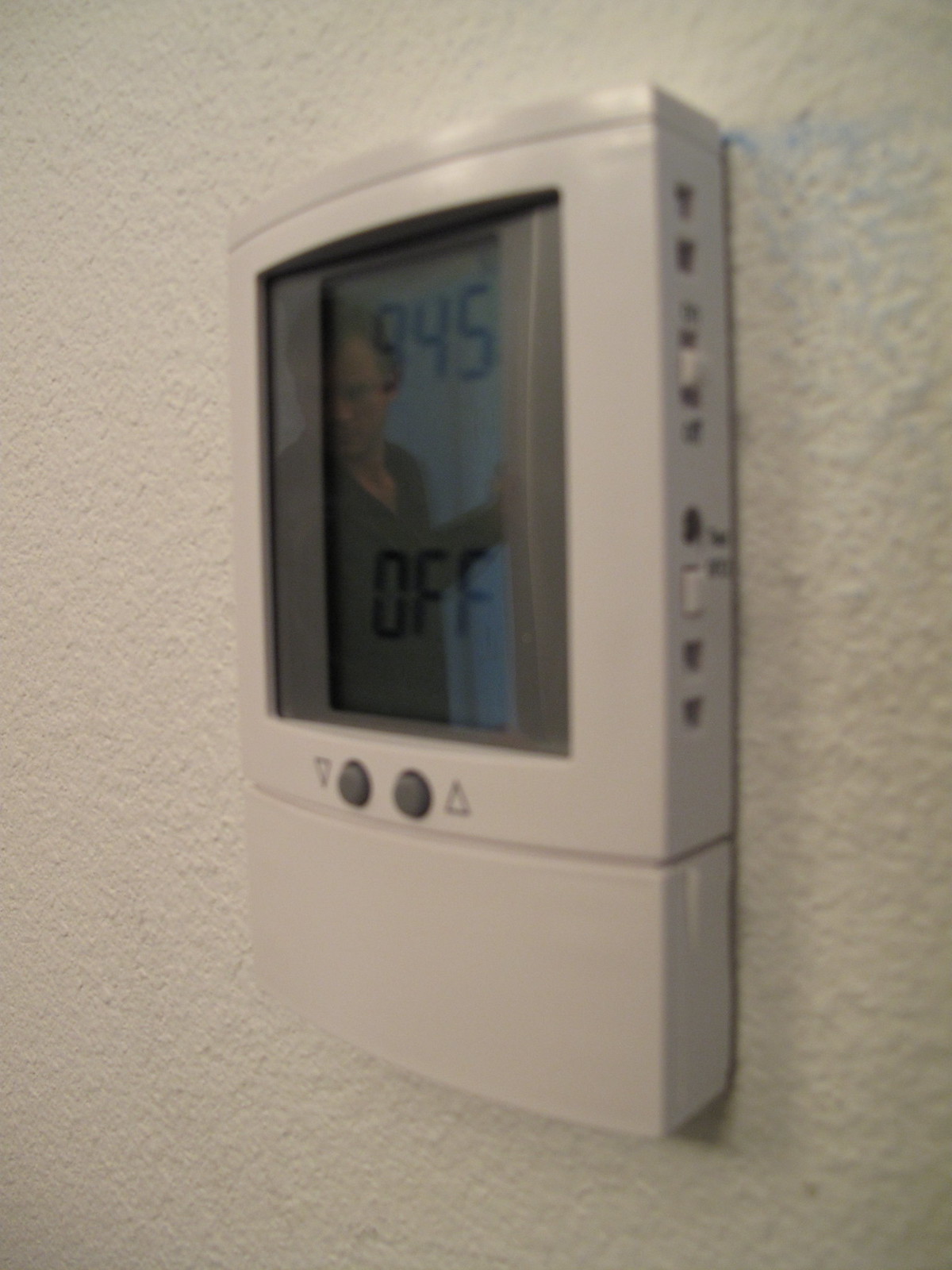The image showcases a square thermostat mounted on a white wall, oriented sideways. The thermostat features a gray digital screen displaying the numbers "945" and the word "OFF" in black text. Along one side of the device are several elements for adjustment: a prominent white switch that can be toggled up or down, a smaller white button positioned below it, and a few small holes. Beneath the digital screen are two small, round gray buttons, each flanked by triangle symbols indicating directions—one pointing downwards and the other upwards.